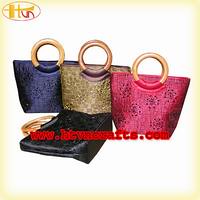This tiny image is an advertisement for a website selling handbags. Displayed against a white background and encased within a pale yellow border, the ad showcases four handbags, each featuring a round handle for carrying. Three bags are standing upright and slightly overlapping, appearing to recede into the background from left to right. The foremost bag is a pink one with some purple patterning. Behind it is a green bag with a snakeskin pattern, followed by a blue snakeskin-patterned bag. A fourth, black bag lies on its side in front of the green bag, with its handle oriented toward the back left and the bottom pointing to the right front of the frame. The handbags have a tote bag structure that is wider at the top than the bottom and seem to have a slightly woven, basket-like appearance. They are adorned with metallic patterns, adding to their stylish look. In the upper left corner of the image, there is a logo in an oval shape with indecipherable yellow lettering. A hard-to-read web address appears in red text across the top of the image. The handle of the black bag, which seems particularly shiny, lies towards the left, and the entire arrangement exudes a chic and artistic vibe.